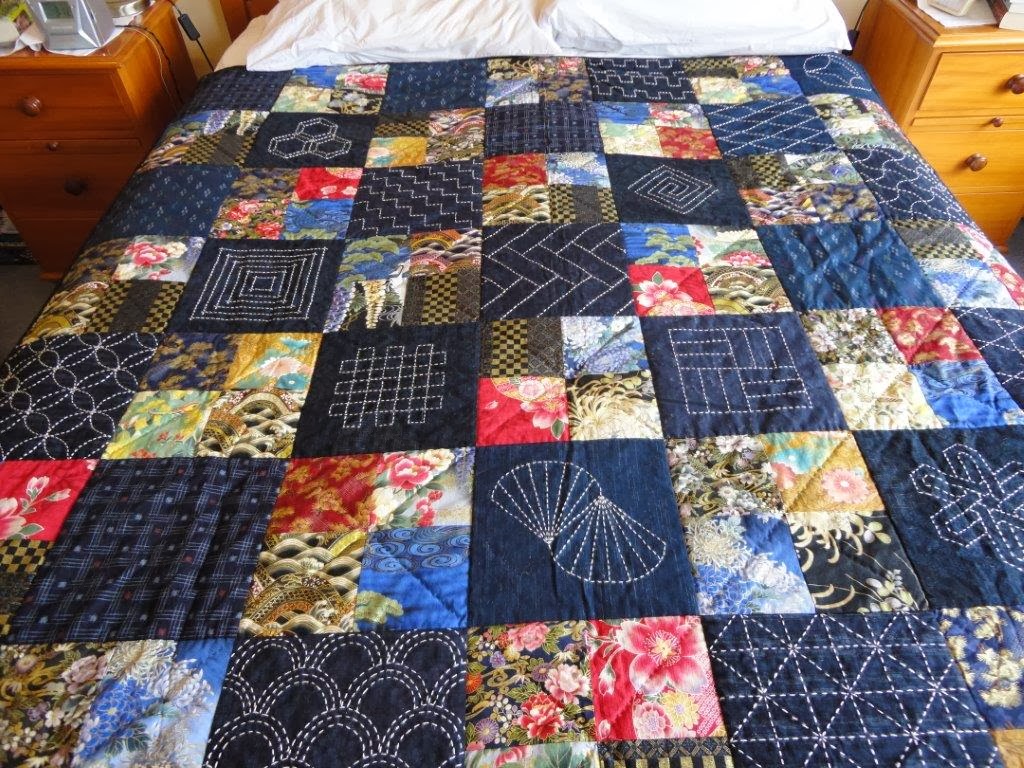In the center of the image, there is a bed adorned with a detailed quilt in various shades of blue, featuring a checkerboard pattern. Each navy square is embroidered with unique designs, including shells, crosshatches, arches, concentric squares, and herringbone patterns. Interspersed among these are squares of printed fabric displaying an array of floral prints with backgrounds in colors such as black, blue, red, and multicolored hues showcasing gold, white, pink, and various flowers. At the top of the bed are white pillows in white pillowcases, adding a subtle contrast with their bearish tint. Flanking the bed are two nightstands; the left one is a darker medium brown, while the right one is lighter brown. These oak night tables each have a couple of drawers, and are set with miscellaneous objects, possibly speakers, boxes, and visible wires extending from them. The composition of the image does not reveal much of the background, focusing closely on the meticulously made bed and its surroundings.